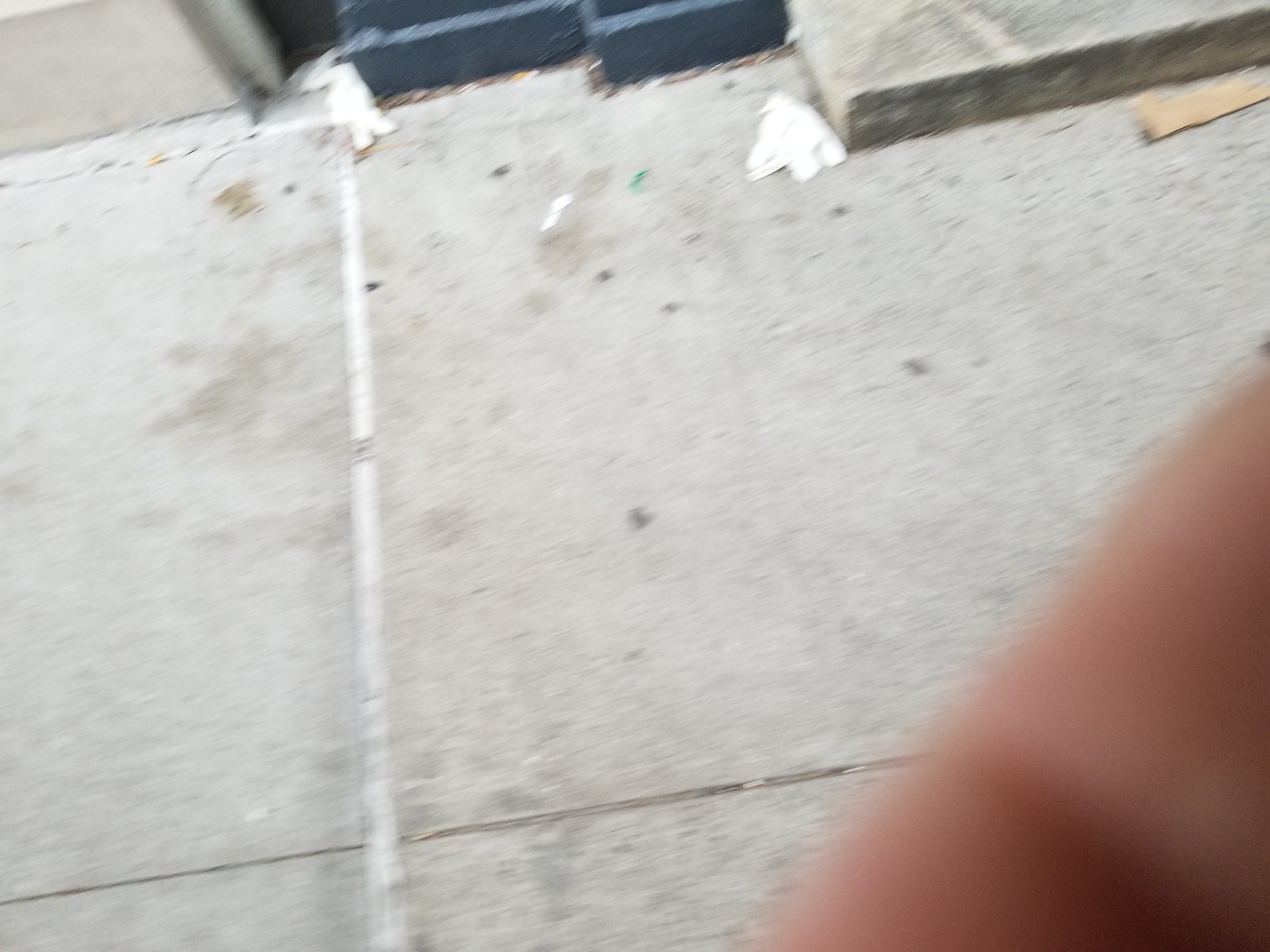The image depicts a blurred close-up of a concrete sidewalk composed of gray slabs with visible stains and dark spots, indicating its slightly worn condition. A prominent white expansion joint runs horizontally, intersecting a filled vertical line, and there are several pieces of litter including white gloves, brown paper, and white paper scattered on the pavement. In the bottom right corner, a fleshy-colored shape, likely the photographer's finger, intrudes into the frame. The scene also features a concrete step leading into a building, along with dark or gray-blue brickwork and molding, suggesting the adjoining building is dark blue. The image captures a snapshot of an urban street, characterized by its mixed and nondescript trash and the surrounding concrete structures.